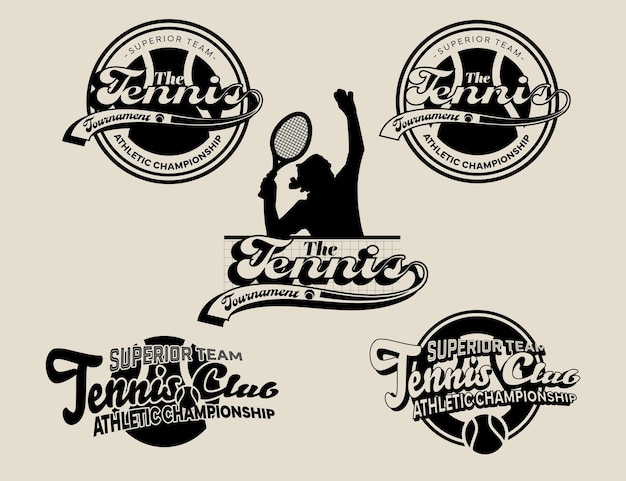This is a computer-generated image representing a tennis tournament, featuring a central silhouette of a man poised to serve a tennis ball with a racket in hand. Surrounding this central figure are four distinct logos placed in each corner. The top left and top right logos share the text "Superior Team," "The Tennis Tournament," and "Athletic Championship," with the top left logo incorporating a unique design where the word "tournament" is elegantly scripted against the tail of an 'S'. The bottom left and bottom right logos also include the phrases "Superior Team," "Tennis Club," and "Athletic Championship," with one of these logos depicted in front of a tennis ball. The entire background of the image is rendered in a light beige color, giving it a refined and elegant aesthetic.